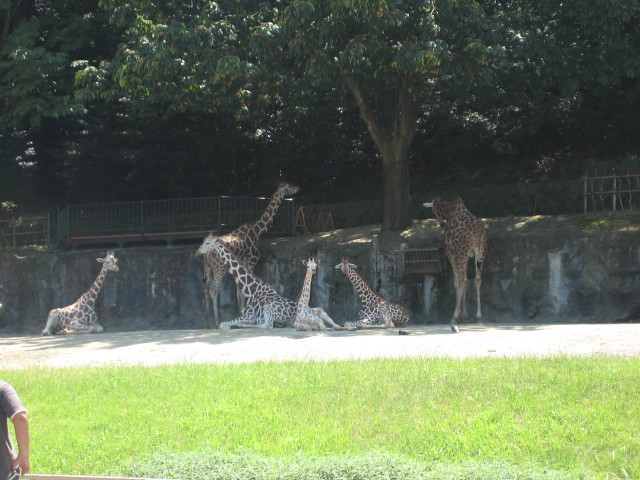This photograph captures a giraffe enclosure at what appears to be a city zoo. In the background, under the shade of dense green trees, a family of giraffes is gathered, some lounging on a flat, sandy area while others are standing. The peaceful scene includes several giraffes: one standing tall and peering over a rock and concrete border lined with a short green fence, another possibly grazing nearby, and multiple others sitting, including two baby giraffes. The enclosure is bordered by a wooden fence, and a hint of a building roof is visible above the trees. The immediate foreground features a vibrant grassy area, with a man's arm and waist just visible—wearing a dark shirt and hand on hip, likely observing the majestic creatures. Additionally, a small waterfall trickles from a rock formation, adding to the serene ambiance of the enclosure.